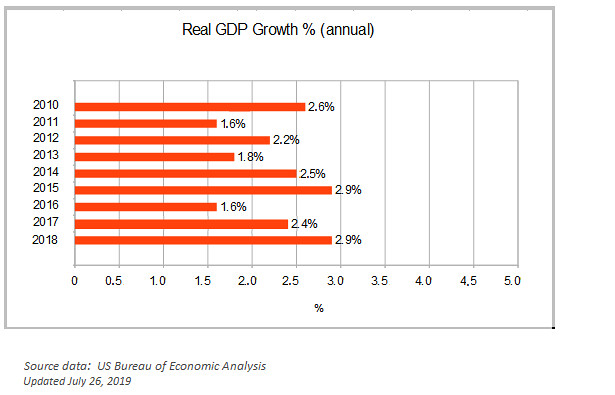The image is a light gray line graph titled "Real GDP Growth Percentage Annual." It displays annual real GDP growth percentages on the x-axis, ranging from 0.0% to 5.0%, and years on the y-axis, spanning from 2010 to 2018. Each year is labeled with its respective GDP growth rate: 2010 at 2.6%, 2011 at 1.6%, 2012 at 2.2%, 2013 at 1.8%, 2014 at 2.5%, 2015 at 2.9%, 2016 at 1.6%, 2017 at 2.4%, and 2018 at 2.9%. The source of the data is the U.S. Bureau of Economic Analysis, with the information updated as of July 26, 2019.